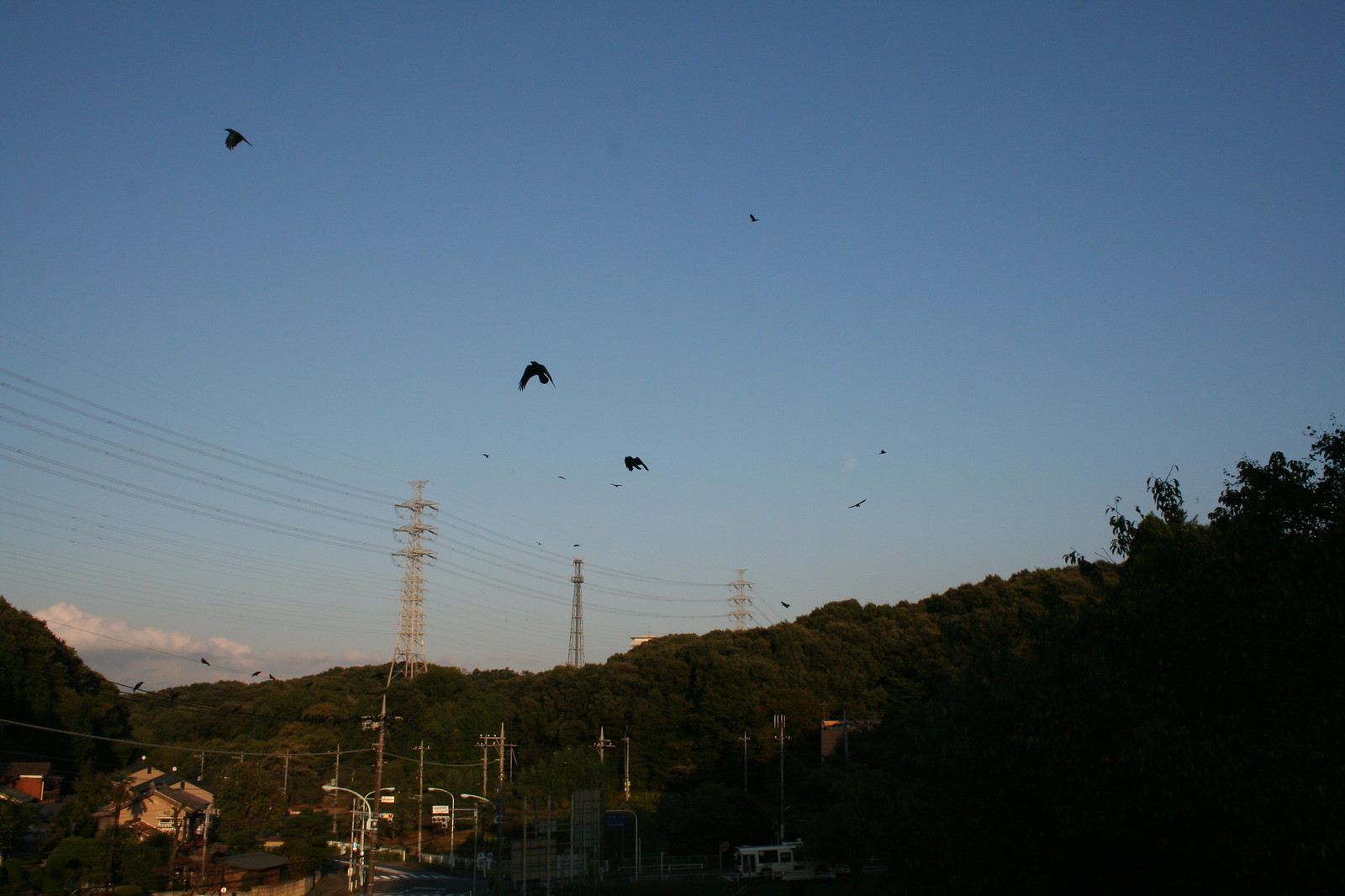The outdoor photograph captures the twilight scene of a village nestled amongst verdant hills and green mountains, with trees and homes shaded in the dimming light. The dark blue sky overhead is dotted with rolling clouds, and amidst the fading sunlight, a multitude of large birds, appearing as black silhouettes, glide across the expanse with their wide wingspans. Dominating the mid-section of the image are several tall power lines, stretching from the mid-left to the mid-right, each strung with three levels of electric wires. Below, the village features streetlights peeking through the shadows, further highlighting the layering of nature and human habitation in this serene landscape.